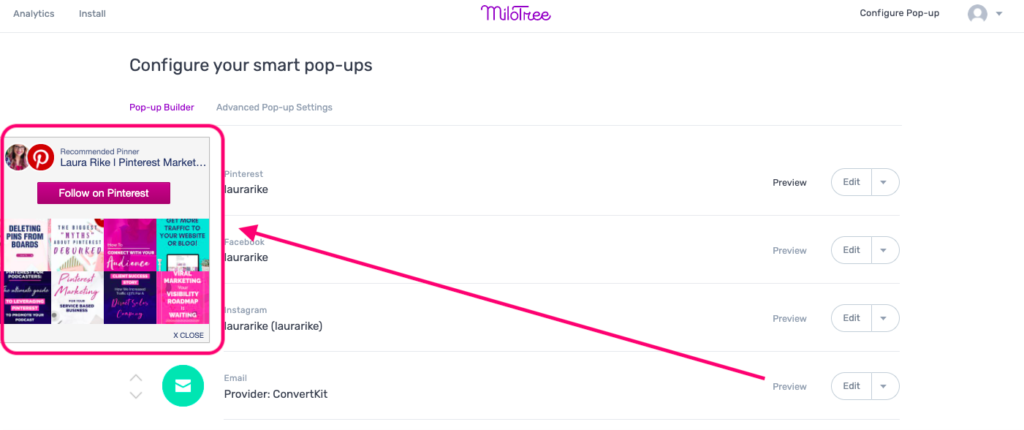This image displays a snapshot of a website with a clean white background. At the top left corner, the options "Analytics" and "Install" are visible. Centered at the top, the site name "MiloTree" is displayed in a vibrant pink-purple hue. On the far right, there's the option to "Configure Pop-Up." Adjacent to this is a drop-down box for the user icon.

On the left side of the image, several tabs are present, including "Pop-Up Builder" and "Advanced Pop-Up Settings." Above these tabs, the heading "Configure Your Smart Pop-Ups" is prominently highlighted in black. A pink-outlined box is expanded on the left, containing a recommendation: "Recommended Pinner: Laura Reich Pinterest Marketing," along with a button to follow on Pinterest. Additional items are listed below this section.

A close button (X) is located at the bottom right of the pink-outlined box. A pink arrow points from the right side of the image to the pink-outlined box, indicating that the pop-up is being previewed. This pop-up preview feature provides users with more information about the pop-up builder functionality.